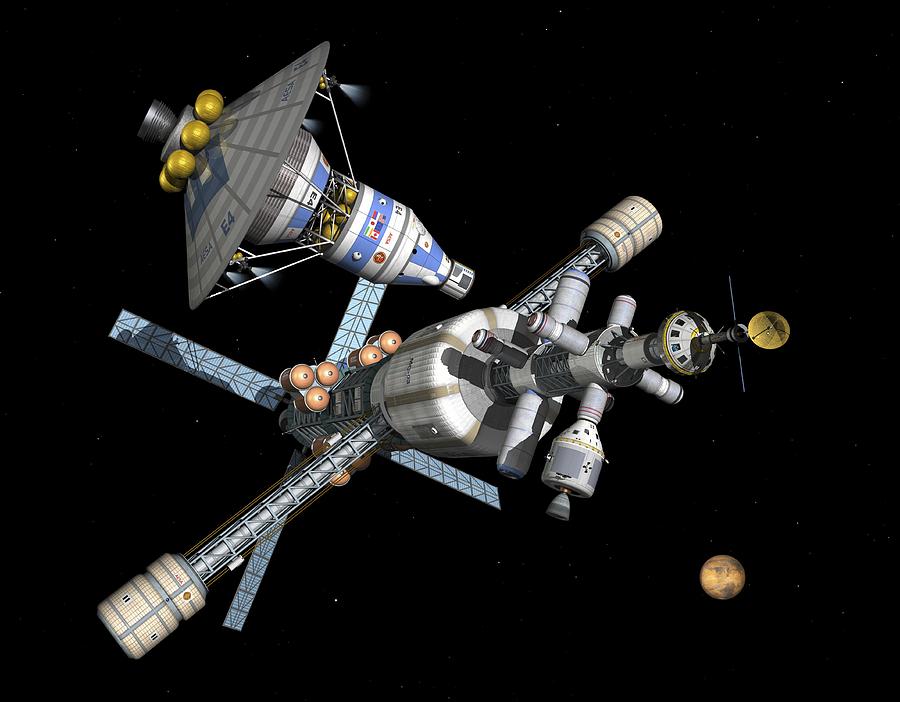The image depicts a sophisticated and intricately designed space station or satellite set against a black, star-sparse background. The structure features interconnected modules adorned with the flags of various countries, including the United States, Japan, and Canada, symbolizing international collaboration. A prominent American flag is seen next to a blue flag, while a Japanese flag is situated above it. The station showcases the identifier "E4" in blue lettering and is characterized by numerous gold spherical elements arranged around its top. These spheres are accompanied by what appears to be a thruster or booster system linked to a series of cylindrical tubes.

One end of the space station is equipped with four windmill-like blades or fan-like extensions, reminiscent of a ceiling fan, hinting at their use for stabilization or power generation. Extending from these blades is a cylindrical segment capped with smaller cylindrical tubes and culminating in a satellite dish, bearing an antenna beneath it.

The lower structure is complex, comprising tubular elements banded with various inscriptions. Sticking out horizontally from this section are two appendages with small white accessories at their ends, possibly for communications or thermal regulation. The backdrop features a planet or a large gold globe, enhancing the outer space context of the image. The overall scene combines elements of both realistic imagery and drawing-like detail, capturing the viewer's imagination with its futuristic and multifaceted design.